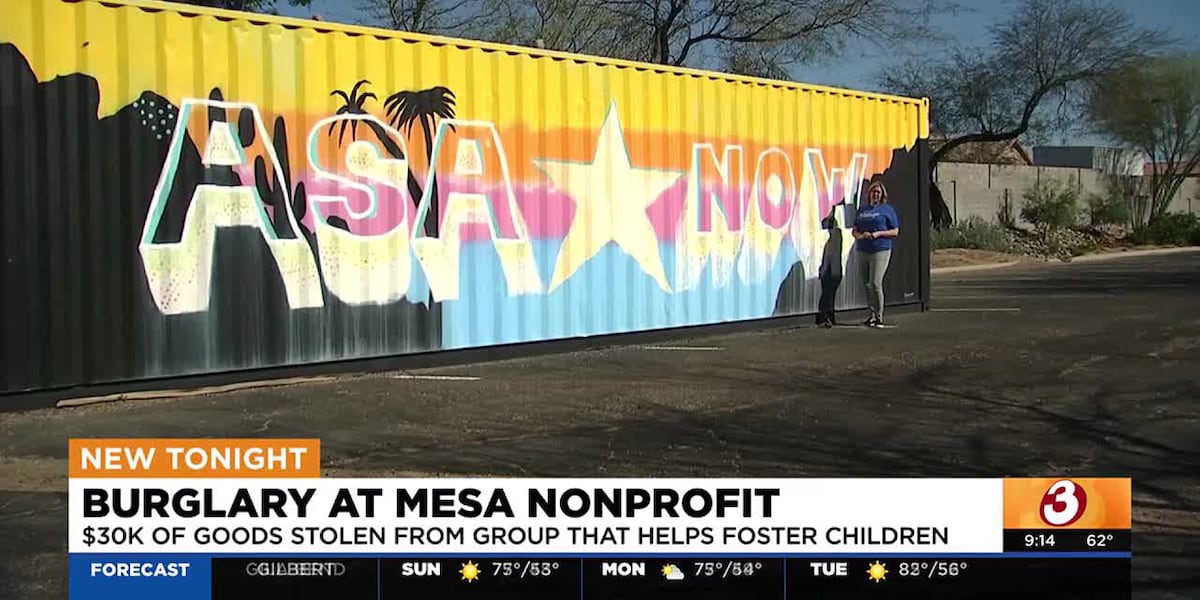The image is a detailed screenshot from a television news program. At the top, there is a small orange rectangular banner with the white text "NEW TONIGHT." Below it, a larger white banner with black text reads, "BURGLARY AT MESA NONPROFIT: $30,000 OF GOODS STOLEN FROM GROUP THAT HELPS FOSTER CHILDREN." To the right of this banner is the news organization's logo, which consists of a large white number "3" encased in a red circle and set against an orange background. Beneath this, a smaller black banner displays the time "9:14" and the temperature "62°."

At the very bottom of the screen, a black banner provides a weather forecast for the following days: "Gilbert Sunday: 75°/53°, Monday: 75°/54°, Tuesday: 82°/56°," with symbols next to the temperatures indicating the weather conditions. 

The main part of the image shows a woman standing next to a brightly painted shipping container. She is wearing grey pants and a blue shirt adorned with blue text. The container itself is yellow at the top, black on the left, and blue at the bottom, with additional orange and pink patterned graffiti. The words "ASA" with a star and "NOW" are prominently displayed in white graffiti-style letters on the container's wall. The background features a parking lot marked by white lines, green trees, a grey wall, some white flowers, and scattered green bushes. There are also buildings visible behind the parking lot, including a tan house with a brown roof and additional structures with grey and orange rooftops.